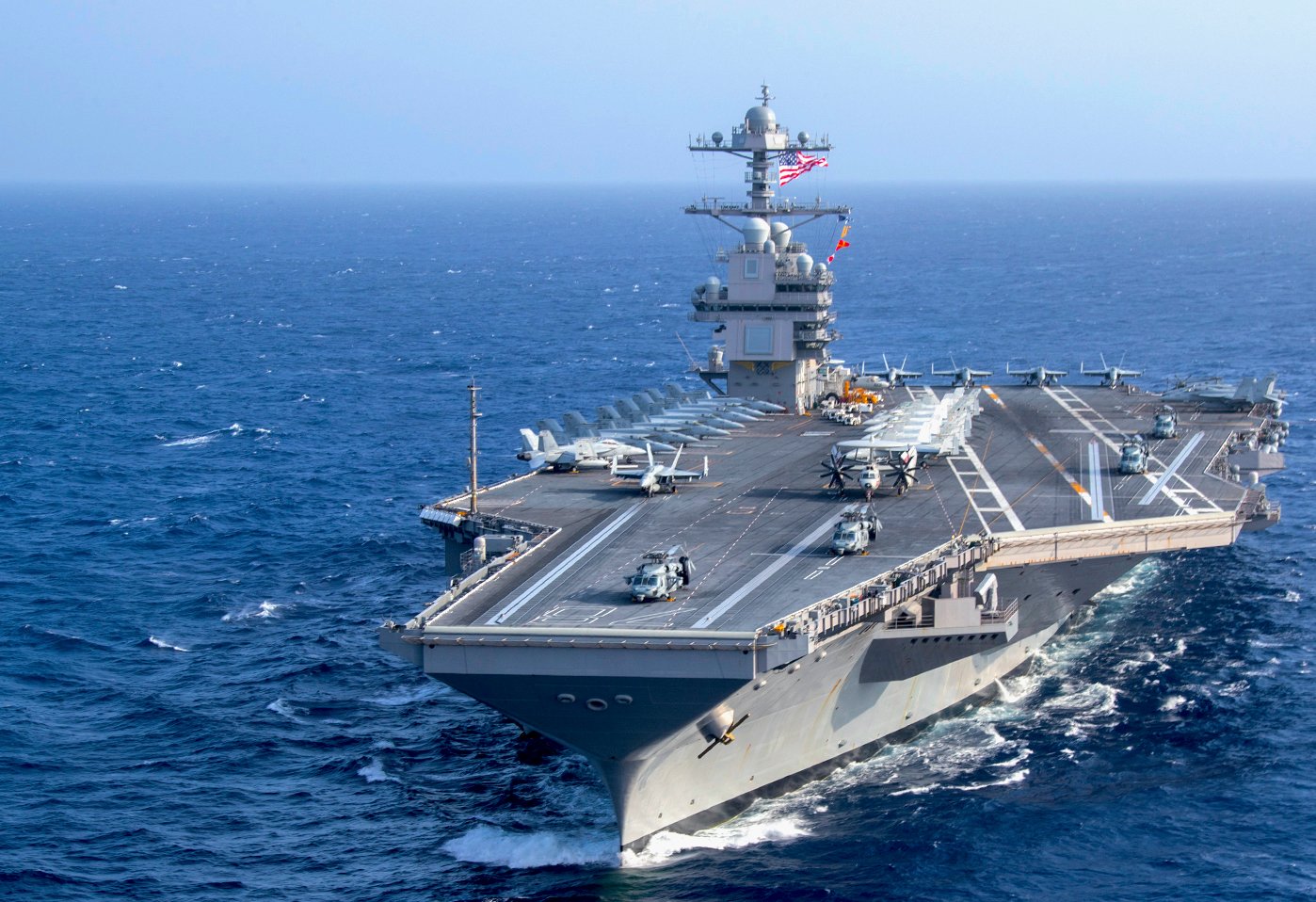In the image, a colossal gray American naval warship, dark with some lighter gray sections, commands the center, sailing smoothly through a vast expanse of clear, very blue ocean under a light blue sky. The top deck of the ship features a runway marked by white lines and an orange and white strip on the right side. On the left side towards the back, ten fighter planes are neatly lined up, accompanied by a few helicopters. The top left of the ship boasts a multi-story tower adorned with an American flag, fluttering amidst a complex web of wires. Two trucks, also stationed on the deck, emphasize the scale and purpose of this imposing war vessel. The ship's movement through the water creates visible white waves, adding to the dynamic scene.